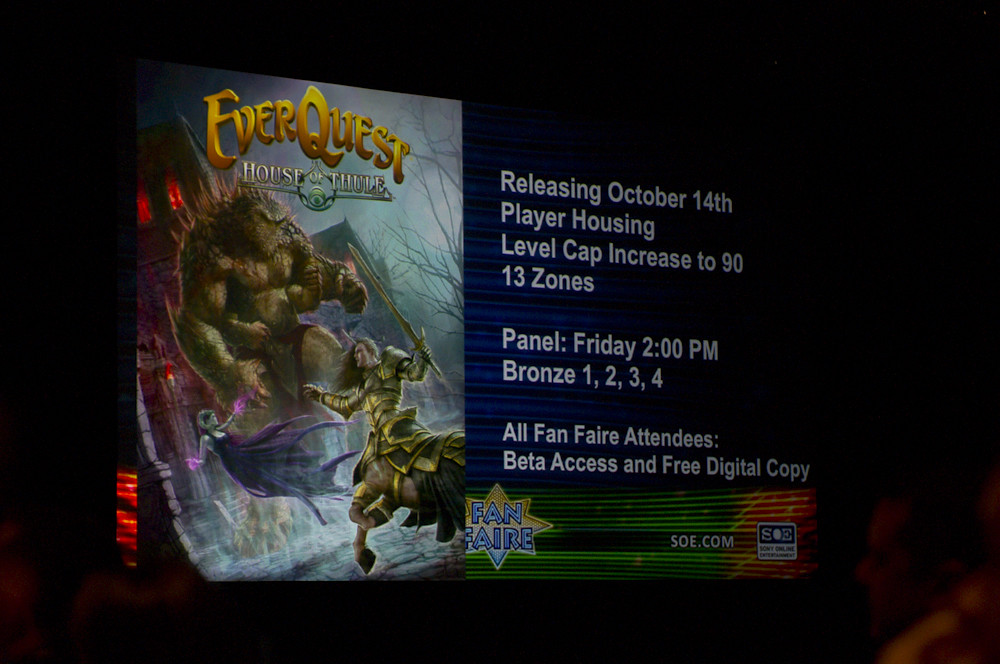The image showcases an advertisement for the EverQuest expansion "House of Thule," likely displayed on a digital screen in a dimly lit room. The centerpiece of the ad features a vibrant illustration depicting an epic battle scene: a monstrous dragon or creature faces off against three heroic figures—a wizardly woman wielding purple and pink magic, a centaur brandishing a sword, and another armored hero. Above this dramatic tableau, the title "EverQuest House of Thule" is prominently displayed in gold letters.

To the right of the illustration, detailed text announces key information: the expansion releases on October 14th, includes player housing with a level cap increase to 90, and introduces 13 new zones. Additional text highlights a panel scheduled for Friday at 2 PM, labeled with "Bronze 1, 2, 3, 4," and notes special perks for attendees of a fan event dubbed Fanfare, including beta access and a free digital copy of the expansion. At the bottom of the advertisement, the SOE (Sony Online Entertainment) logo is visible, with the URL "soe.com" listed beneath it. In the lower right corner of the ad, a faintly visible, reddish-lit shadow of a person's face hints at the dark setting in which the sign is displayed.